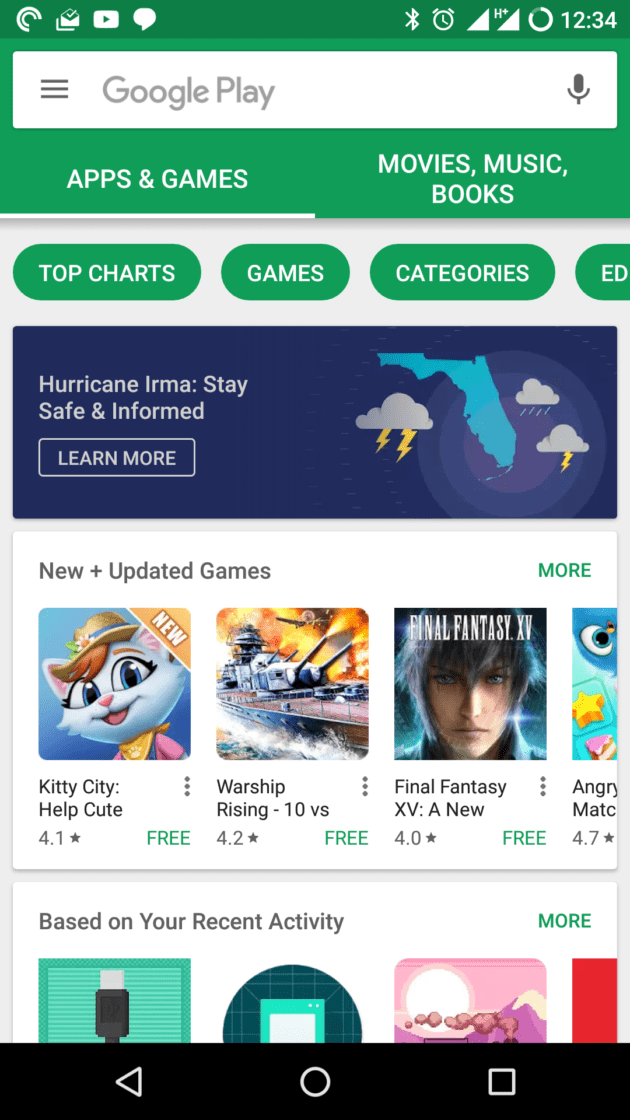The phone screen displays a variety of notifications and app interfaces:

- **Top Section**: 
  - **Notification Bar**: Shows the time as 12:34. Icons indicate that you have new mail, a YouTube notification, a text message, Bluetooth is enabled, an alarm is set, and there is cellular signal strength represented by bars.
  - **Google Play Search Window**: A white search bar with gray text, featuring two navigation tabs – 'Apps & Games' and 'Movies, Music, Books.'

- **Main Content Area**: 
  - **Tabs**: Under a green header with white text are tabs labeled 'Top Charts,' 'Games,' and 'Categories.' Another tab appears partially cut off, displaying 'ED.'
  - **Hurricane Alert**: A notification about Hurricane Irma with the text "Stay safe and informed. Learn more" on a blue button with white text. An illustration of the state of Florida in blue with three clouds, lightning, and rain is shown beneath it.
  - **New & Updated Games**: This section features a list of games with brief descriptions, ratings, and availability:
    - **Kitty City**: Described as "cute," rated 4.1 stars, and free.
    - **Warship Rising**: Noted as a 10-player versus game, rated 4.2 stars, and free.
    - **Final Fantasy XV**: Mentioned with a 4.0-star rating and free.
    - Additional game titles and descriptions are cut off midway down the screen.

This is a detailed depiction of a phone screen showcasing various app notifications, alerts, and recommended game listings.